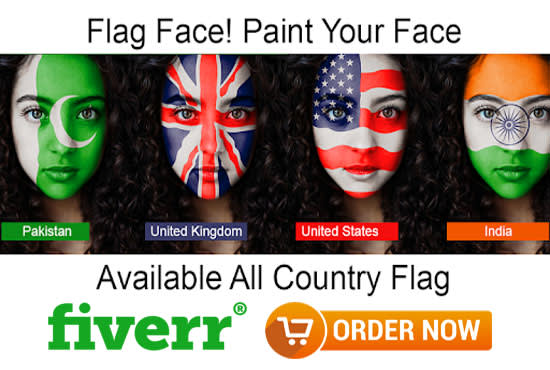This advertisement for Fiverr showcases its face-painting services, featuring a central image of a girl with curly hair whose face is painted in four different national flags. Starting from the left, her face is painted with the Pakistani flag, featuring a white vertical stripe on the left third and a green section with a crescent moon covering the rest. This face is labeled "Pakistan" with a green background and white text. 

Next is the United Kingdom flag, depicted with red and white stripes forming crosses on a blue background, labeled "United Kingdom" on a blue background. The third face shows the United States flag, with a blue rectangle filled with white stars over her right eye and red and white stripes across the rest of her face. It is labeled "United States" on a red background. The final face displays the Indian flag with orange across the forehead, white in the middle section, and green at the bottom, along with a blue Ashoka Chakra in the center. This is labeled "India" on an orange background.

At the top of the advertisement, black text reads "Flag Face! Paint Your Face." The bottom mirrors this with the text "Available All Country Flag" in black. To the lower right, the green Fiverr logo with a registered trademark appears alongside an orange "Order Now" button with a shopping cart icon.